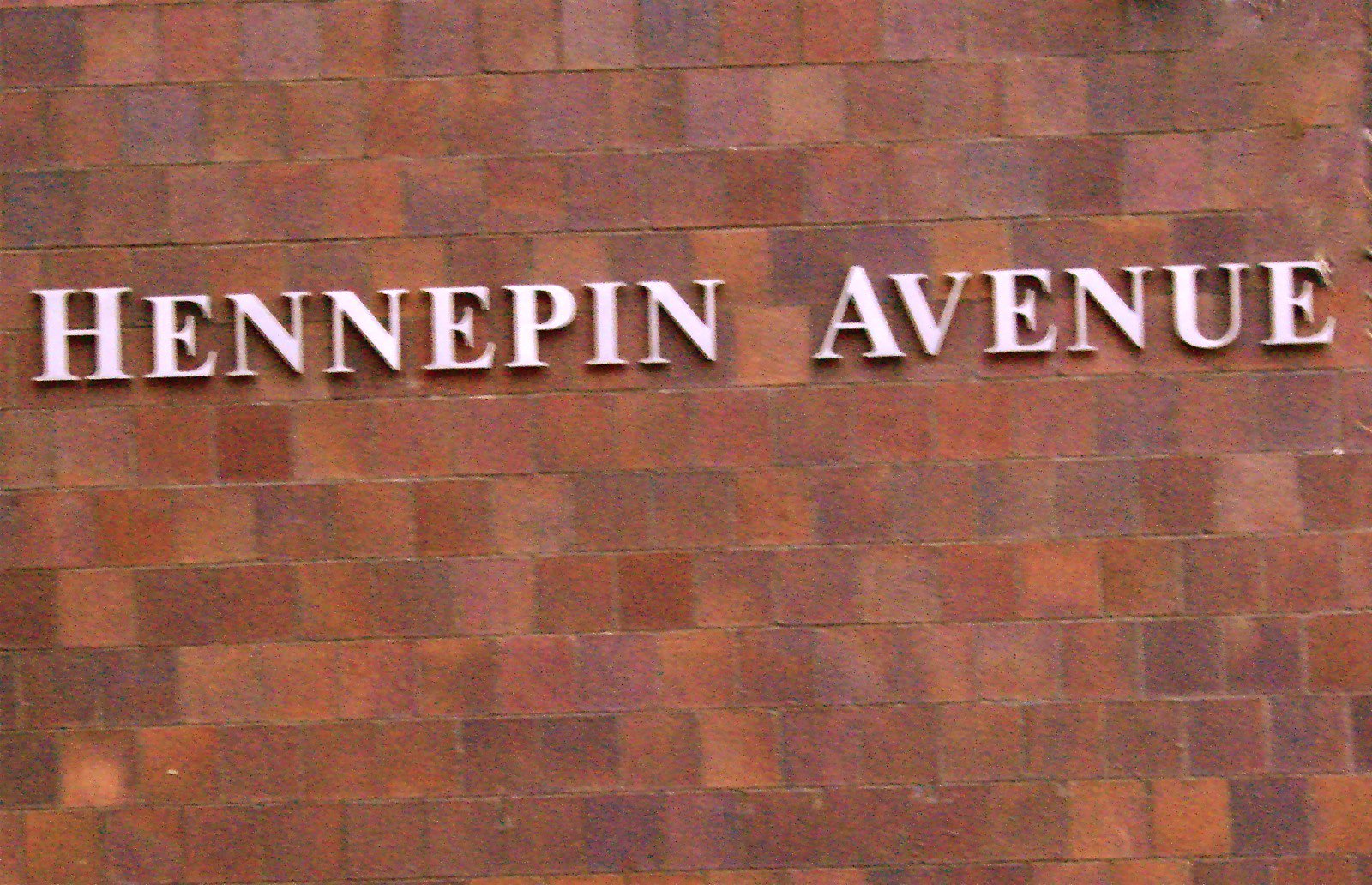The photograph captures an intricately designed wall on Hennepin Avenue, one of the main and most vibrant streets in Minneapolis, Minnesota. The wall features an eye-catching, colorful square brick pattern. Each brick, laid with its short end out, creates a tapestry of hues that almost resemble decorative tiles. Mounted on this multicolor backdrop are light-colored gray metal letters that spell out "Hennepin Avenue" in a square font, adding a sleek, modern touch to the historic thoroughfare. Known for its lively atmosphere and eclectic charm, Hennepin Avenue stands as a bustling, slightly wild, yet quintessential part of the Minneapolis landscape.